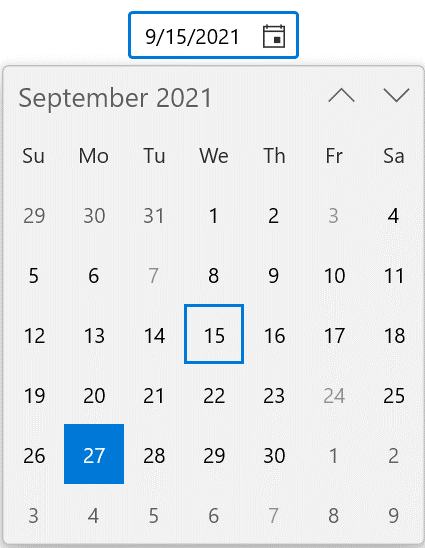Here is a detailed and polished caption for the provided image:

---

This image is a screenshot of a digital calendar display for the month of September 2021. At the top, there is a small rectangle with a thin blue border, inside which the date "9/15/2021" is prominently shown next to a calendar icon. Below this, the current month and year, "September 2021," are displayed in bold black letters. To the right of this text, there are two arrowheads for navigation: the upper arrowhead points upwards, and the lower arrowhead points downwards, indicating controls to navigate between months.

The calendar layout features seven labels that represent the days of the week, each abbreviated to two letters: "SU" for Sunday, "MO" for Monday, "TU" for Tuesday, "WE" for Wednesday, "TH" for Thursday, "FR" for Friday, and "SA" for Saturday. The week starts with Sunday as the first day. 

In this calendar, the month of September 2021 begins on a Wednesday, marked by "WE" and includes all the dates from the 1st to the 30th. The last day of the month, the 30th, also falls on a Thursday. The calendar grid comprises six rows (weeks), with the days outside the September range grayed out, emphasizing that only the dates from September 1st to September 30th are bold and prominent.

---

This caption offers a clear and thorough description of the calendar's structure and visual elements.